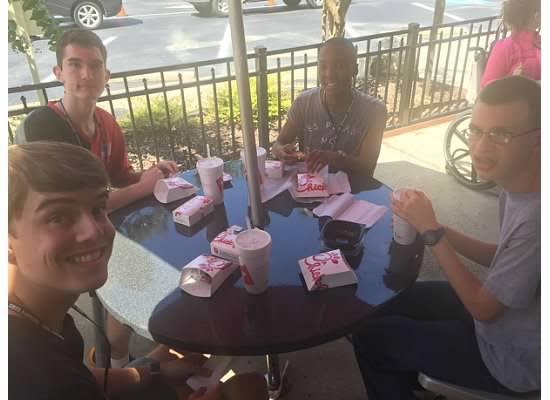In this lively outdoor scene, four young men are seated around a round patio table at a restaurant, enjoying a meal on a sunny day. The setting is vibrant, with a street and a couple of parked cars visible in the background. 

In the lower left of the image, a young man with brown hair is caught mid-turn, beaming at the camera. Directly above him, another young man with brown hair, clad in a mostly red shirt and sporting a lanyard around his neck, gazes into the camera lens.

At the top right of the table sits a smiling African-American young man with a lanyard bearing blurry text around his neck. He is wearing a gray short-sleeve shirt, adding to the casual atmosphere. Lastly, in the lower right corner, a young man with short brown hair and glasses looks directly at the viewer, a watch on his left wrist.

The table in front of them is bustling with activity, adorned with boxes of food and drink cups clearly marked with the red Chick-fil-A logo. 

Adding to the depth of the scene, another person clad in a pink top, seated in a wheelchair, is visible at a neighboring table to the far right. A fence runs along the background, neatly separating the dining patio from the street and sidewalk areas, framing this cheerful gathering.